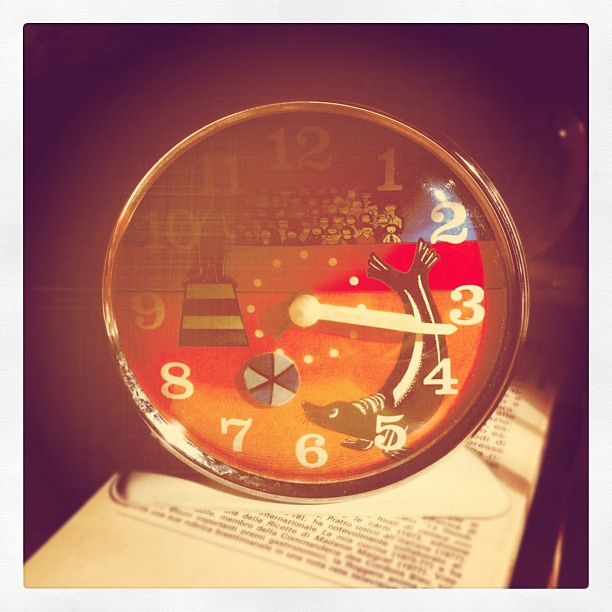This square image captures an eye-catching alarm clock resting atop a printed paper scattered with text. The scene is bathed in soft sunlight streaming in from the lower right corner, casting a delicate illumination on part of the clock's face while leaving the rest in shadow. The alarm clock is adorned with a gold bezel and features a whimsical face characterized by a vibrant color palette of blue, red, and white. It showcases a charming nautical theme, with a lighthouse, a beach ball, and a seal cheerfully interacting before a crowd, all artistically arranged against a backdrop formed by the red band between the white and dark blue sections. The clock's numbers are presented in stylized Times Roman font, with Roman numerals from one to twelve circling the dial. The white hour and minute hands stand out clearly against the colorful face, indicating the time as seventeen minutes past three. This image beautifully merges practical design with playful details, creating a visually engaging and detailed snapshot.